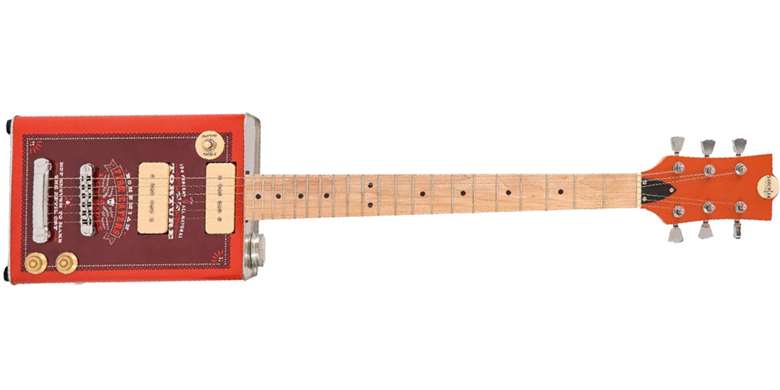This is a detailed description of a unique, handmade six-string guitar. The body is constructed from an old-style oil can that is red-framed, with a dark purple center. The oil can, which is oriented on its side, holds all the essential guitar components. In the center of the can, multiple silver metallic pieces are bolted on to secure the strings, which extend up to a light-colored, ash wood fretboard attached to the top of the can. The headstock, also red, features six silver tuning knobs. The oil can's body includes additional functional elements such as golden dials, a chrome dial, and a power switch. There are illegible small texts on the can, adding to its vintage aesthetic. The overall setup includes elements like metallic circles and square shapes. The photograph is taken against a plain white background, highlighting the guitar's visually striking contrast of red, purple, and metallic colors.